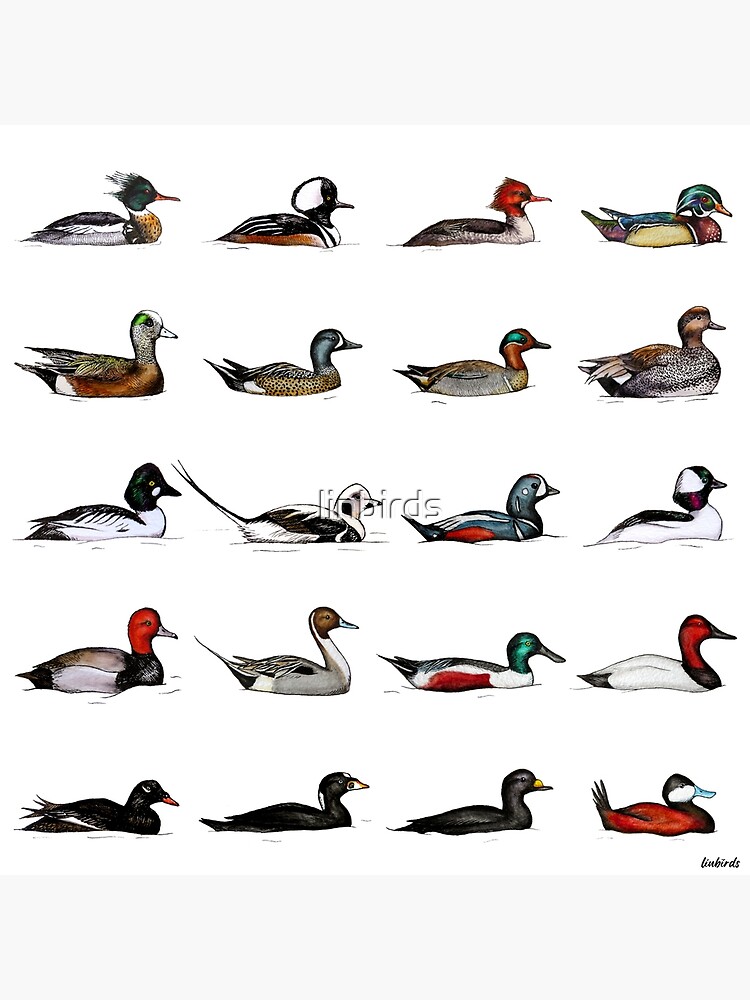This is a square, computer-generated or colored drawing featuring an evenly spaced grid of 20 ducks, arranged in five rows of four against a plain white background. Each duck in the image represents a different species or design, showcasing a variety of colors including red, green, black, gray, and blue. The ducks are depicted from a side view, all facing the same direction, and are uniformly sized. The design appears minimalistic, likely sketched with an ink pen. In the center of the image, there is a subtle watermark that reads "Lynnbirds" in light gray text, indicating the creator or copyright owner of the artwork. The intricate details of the ducks include diverse head and body patterns, ranging from solid to striped and even zebra-like designs.